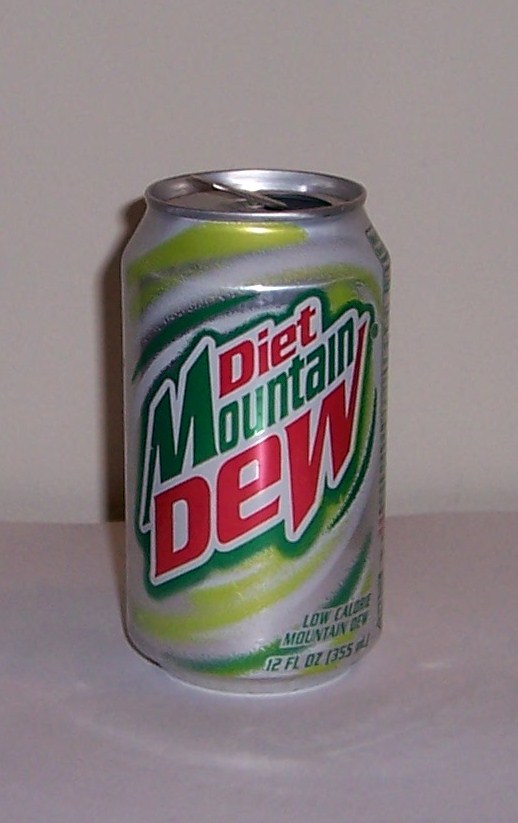This is a detailed color photograph of an opened 12-ounce Diet Mountain Dew can in portrait orientation. The silver metal can features the classic Diet Mountain Dew logo with 'Diet' in red, 'Mountain' in green, and 'Dew' in red against a backdrop of lime green swirls and dark green accents. The tab at the top is partially raised, revealing the black void where the metal tab has been broken out. The bottom of the can states 'Low Calorie Mountain Dew' in dark green text and '12 FL OZ (355 mL)'. The can rests on a light reddish-pinkish-brownish surface that appears to be stone, marked with white spots and darker patches suggesting uneven toning. In the background, a beige wall casts a shadow to the left of the can, highlighting the contours of the can including the lip, slightly diagonal midsection, and the vertical body of the shadow. A glimpse of the nutritional label can be seen on the far right side of the can.